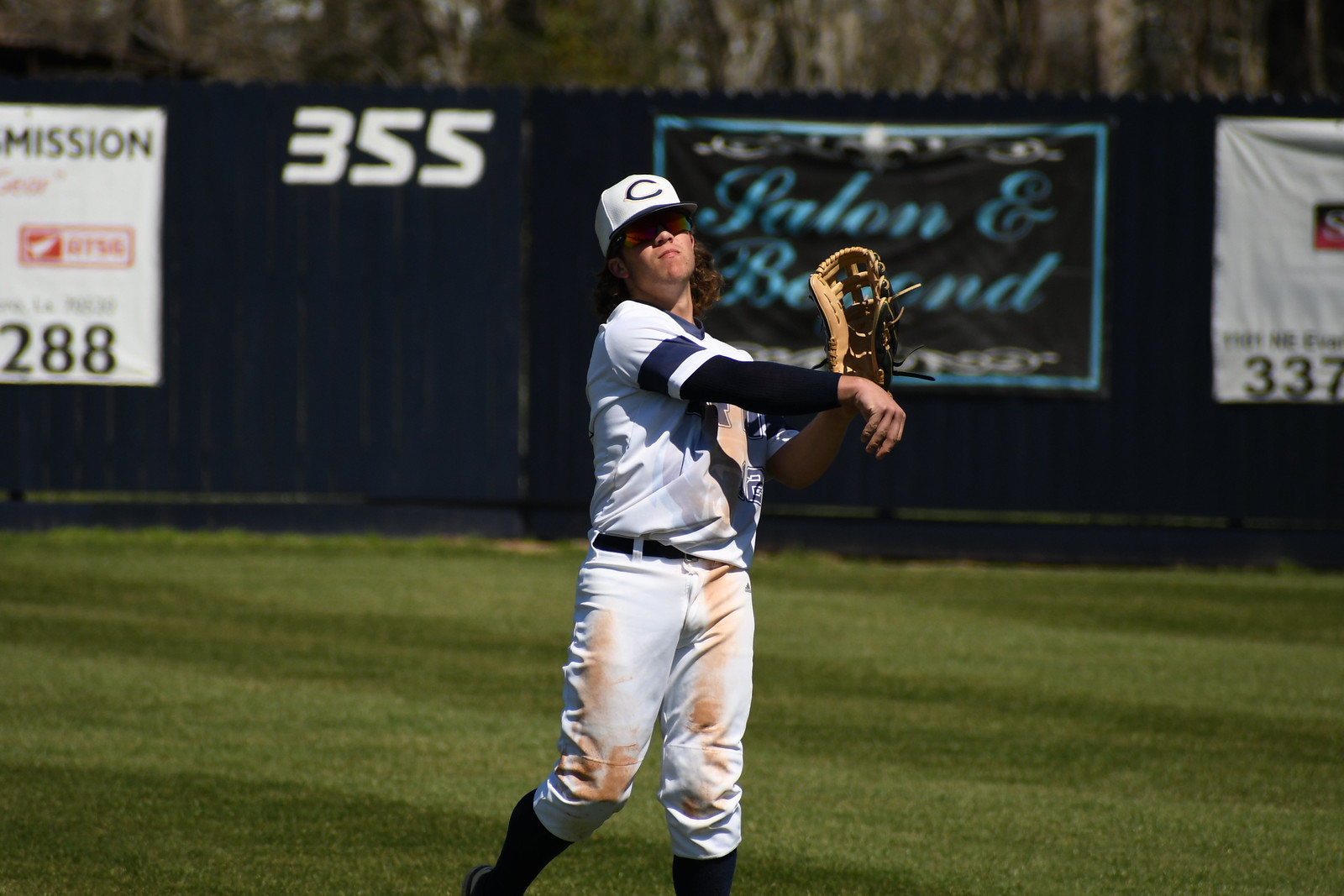A baseball player stands poised in the outfield, captured mid-throw with his right arm extended and his left hand gripping a mitt. He wears a white uniform accented with dark blue—the top is white with long blue sleeves reaching his wrists, while his pants are white with a blue belt and knee-length blue socks. His cap, also white, features a blue "C" logo, and under its brim, he appears to be wearing glasses as he gazes upward with a neutral expression. His uniform shows signs of a recent head-first slide, marked by dirt on the front. In the background, neatly mown grass in alternating dark and light green stripes stretches toward a dark navy fence adorned with colorful advertisements, some partially obscured. The visible ads include fragments of text like "salon" and "beyond," and the number "355" marks the outfield distance. Beyond the fence, the image softly transitions into blurred foliage and hints of the sky.